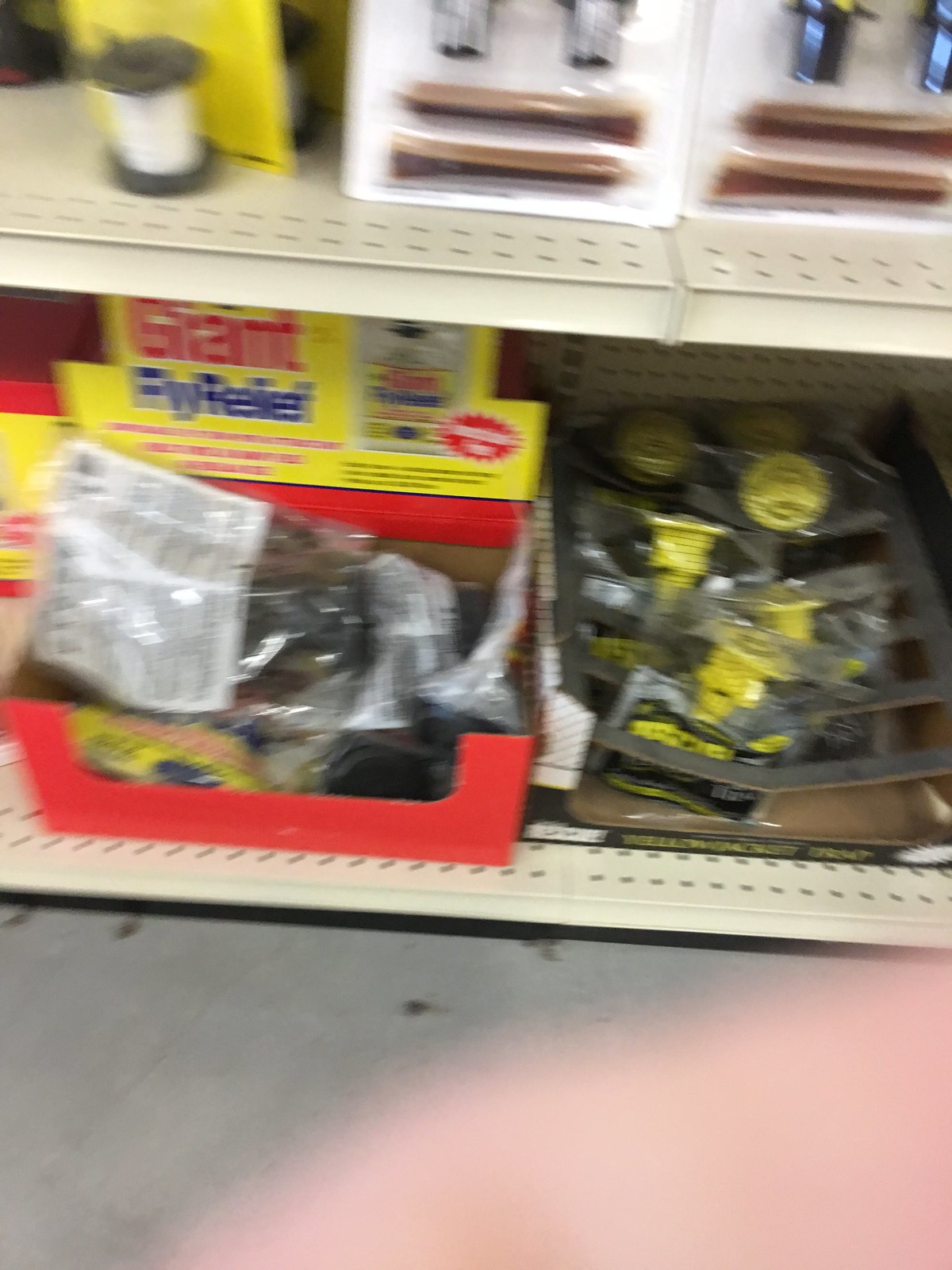The image captures a slightly blurred, out-of-focus interior of a hardware store, focusing on two metal shelves with a tan hue. The lower shelf prominently features a yellow sign with red and blue lettering, possibly indicating the brand "Giant" or "Grant", alongside packaged items, potentially black and yellow traps for capturing flies or bees. To the right of this section is a product that appears to be coiled with a yellow backing and black ends, likely a spool of some sort. Just above these, on the upper shelf, are packages containing what look like tan stakes or metallic and crystal-clear drawer handles. Additionally, there is a white package above resembling small tool handles or drill bits. The bottom right corner reveals a faint blur, possibly from a finger in the frame, and the floor appears somewhat dirty with visible debris.